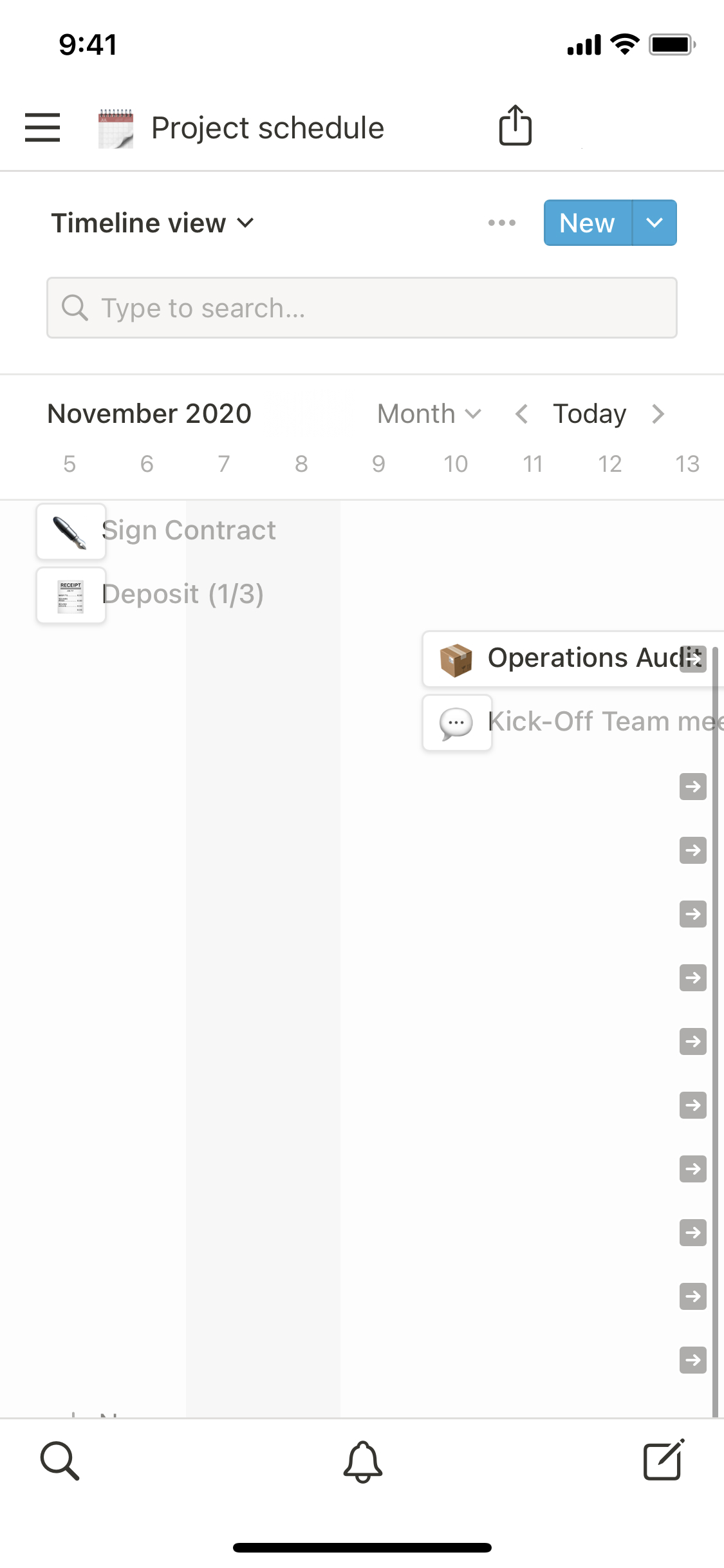The image shows a screenshot of a project management or scheduling app displayed on a smartphone. The time on the device is 9:41. The project currently being viewed is titled "Project Schedule." Prominently featured at the top are icons for menu and share options, as well as the app's logo.

In this particular view, the interface is set to the 'Timeline View,' which can be altered using a drop-down menu. A search bar is visible, allowing users to type and search for specific tasks or events. Beside the search bar, a button labeled "New" with an accompanying drop-down arrow facilitates the addition of new tasks or events.

The calendar in the screenshot is configured to show November 2020, with the current day distinctly highlighted as "Today." Specific tasks and events are displayed with unique icons for easy identification: a signed contract is represented by an icon of a pen and document, and the first deposit out of three is denoted by an icon of a receipt. Upcoming events are also outlined, including an "Operation Audit" symbolized by a box icon and a "Kickoff Team Meeting" indicated by a speech bubble icon.

The bottom navigation menu features icons for search, notifications (signified by a bell), and an edit option depicted as a pencil icon. Overall, the image showcases a clean and well-organized interface designed for effective project schedule management.